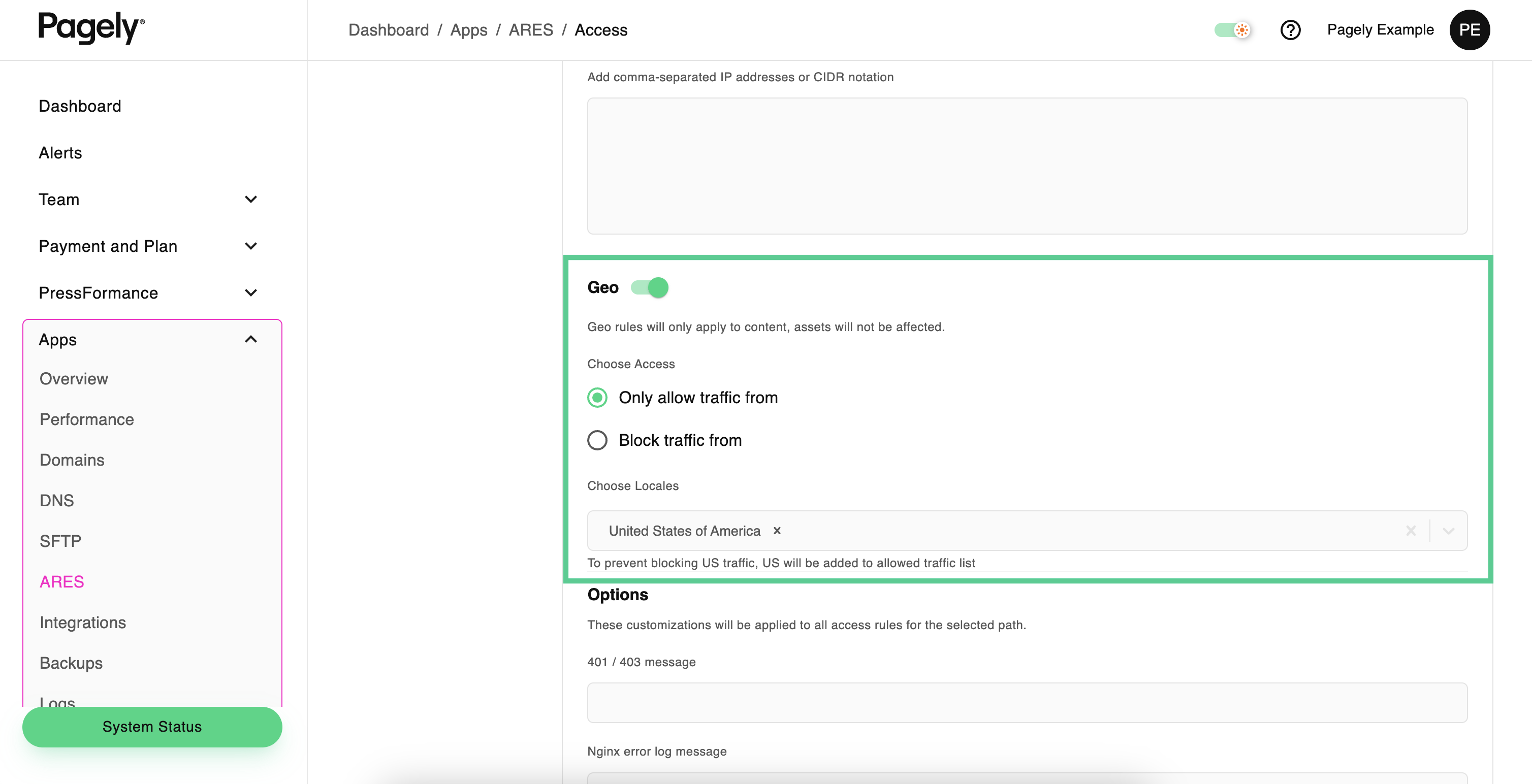**Pagely Landing Page Overview**

The landing page features the user profiles prominently. At the top right corner, "Pagely" is displayed as the site name. In the upper left corner, the label reads "Pagely Example," with an option to toggle P-E on or off.

The navigation menu on the left side includes the following sections:
- Dashboard
- Alerts
- Team
- Payment Plan
- Pressformance (a play on words combining "press" and "performance")
- Apps Overview
- Performance
- Domains
- DNS & SFTP
- ARES (access control)
- Integrations
- Backups
- Logs
- System Status

In the central section of the page, under "Dashboard" and "Apps," there's an ARES access control field where users can add comma-separated IP addresses or CIDR notations. Additionally, there are options for geo-restricting traffic, including "Allow traffic from" and "Block traffic from" specific regions.